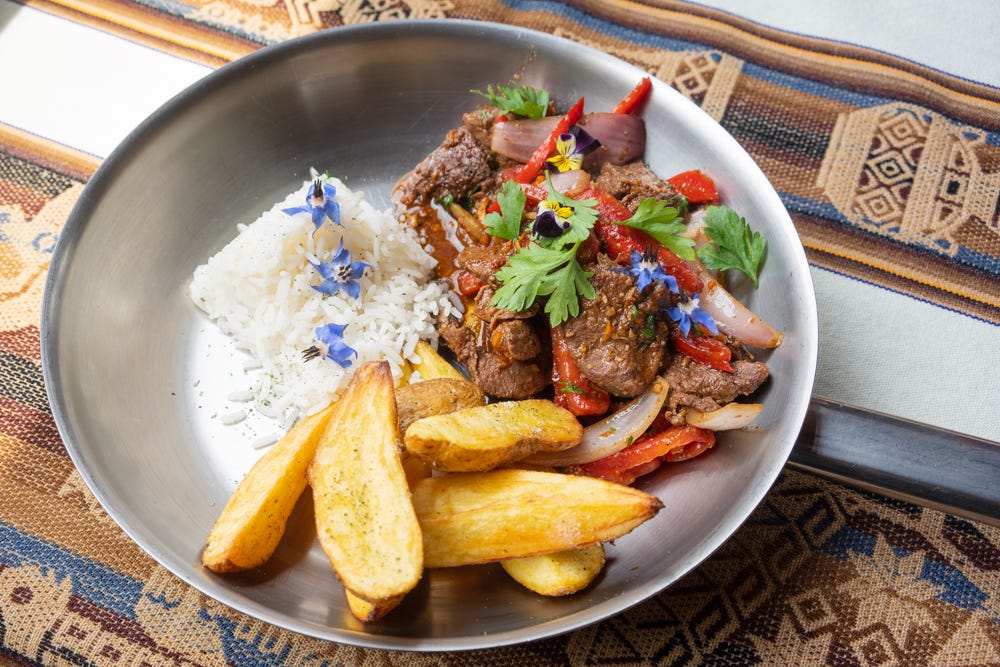This image showcases a detailed, close-up view of a delicious meal presented in a silver metal bowl. The bowl, centrally located, is placed on an intricately embroidered table runner adorned with stripes of blue, brown, black, and rust, as well as decorative patterns resembling vases and snowflakes. Inside the bowl, on the right side, there's a savory beef stir-fry mingled with red peppers, onions, shallots, parsley, and adorned with small blue flowers. To the left of the stir-fry, there's a neat mound of white rice, also embellished with three small blue flowers, adding a touch of elegance. In the front of the bowl, thick-cut steak fries, golden and crispy, made from real potatoes, complete the meal. The colors in the image are vibrant yet harmonious, featuring grays, whites, greens, reds, golden tones, and soft tans. This photograph would likely be used to illustrate a recipe for a beef stir-fry with French fries and rice on a culinary website.